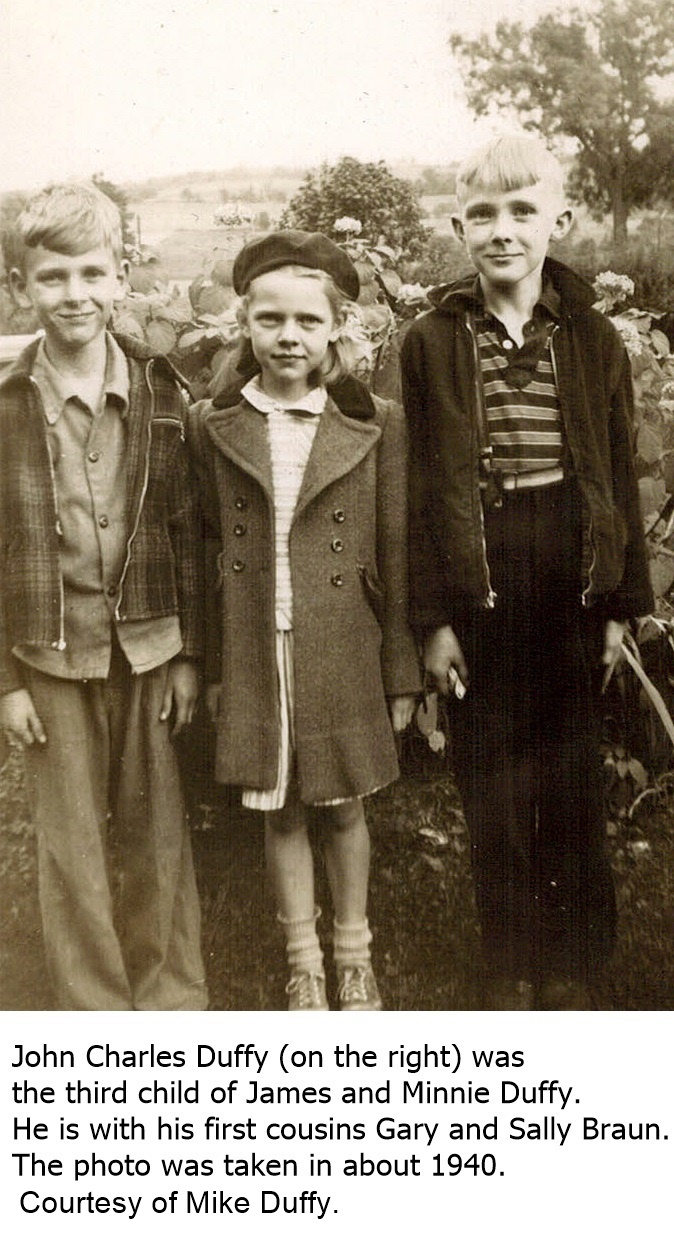This is a detailed black-and-white photograph taken around 1940 in a grassy, country setting with trees and possibly mountains in the distance. The image features three children in the foreground: two boys and a small girl standing between them. The boy on the left is wearing a plaid jacket over a collared shirt and a t-shirt, with short hair. The girl in the center is dressed in a coat and a beret, along with a dress and ankle socks with shoes. The boy on the right, identified as John Charles Duffy, who has short blonde hair, is wearing black pants, a black jacket, and a striped shirt with buttons. John Charles Duffy, the third child of James and Minnie Duffy, stands with his first cousins, Gary and Sally Braun. The photo, courtesy of Mike Duffy, offers a nostalgic glimpse into their family history.